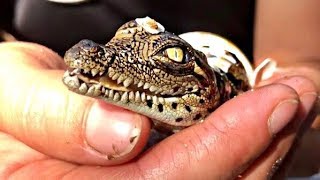This up-close photograph captures a European descent man's cupped hand gently cradling a newly hatched baby crocodile. The man’s hand, featuring short nails and thick, dirt-streaked fingers, contrasts with the hatchling's delicate appearance. The tiny crocodile, adorned with bits of eggshell on its head, boasts a scaly, brown and tannish head with a distinct snout. Its wide, yellow-green eye and rows of tiny teeth are clearly visible, suggesting an alert and curious demeanor. Behind the crocodile, remnants of the eggshell draw attention to its recent emergence. The person holding the hatchling wears a black T-shirt, cradling the baby reptile with care.